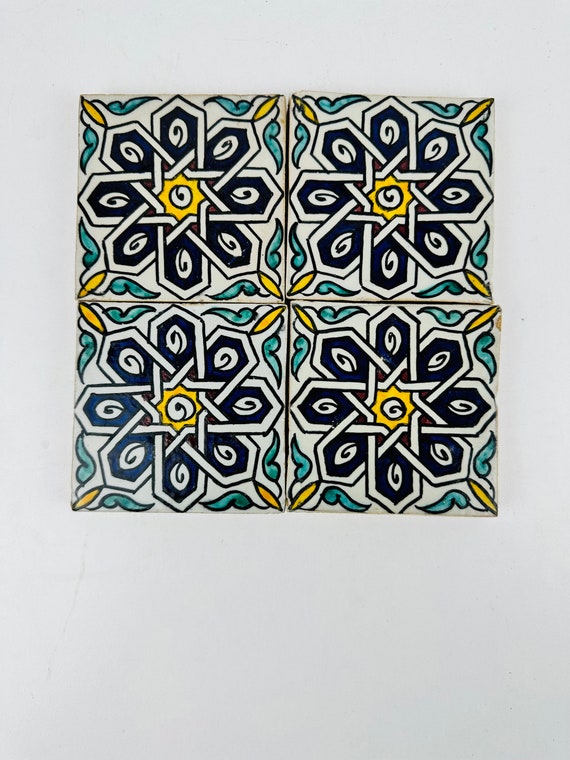This vertically aligned rectangular image consists of a set of four nearly identical graphic panels, arranged in a two-by-two grid, against a light gray background. Each panel exhibits a complex design featuring intricate, pointed shapes resembling tapered rectangles or bookmarks, oriented to form a cross-like pattern. There are eight pointed elements in each panel, with two positioned diagonally and two oriented left-to-right. These shapes have a dark blue interior and a white exterior, interspersed with small white ovals. Centrally, within each cross, lies a yellow area hosting a black and white swirling pattern.

Surrounding the cross-shaped figures are curved, plant-like motifs: yellow ovals at the corners with green, peapod-like shapes extending from them, appearing to have been colored with crayon or colored pencil to create a textured look. The combination of yellow petals with green accents lends a floral aesthetic that contrasts with the geometric precision of the central figures. The overall composition conveys a blend of natural and abstract elements, resulting in a visually stimulating and balanced artwork devoid of any textual elements.